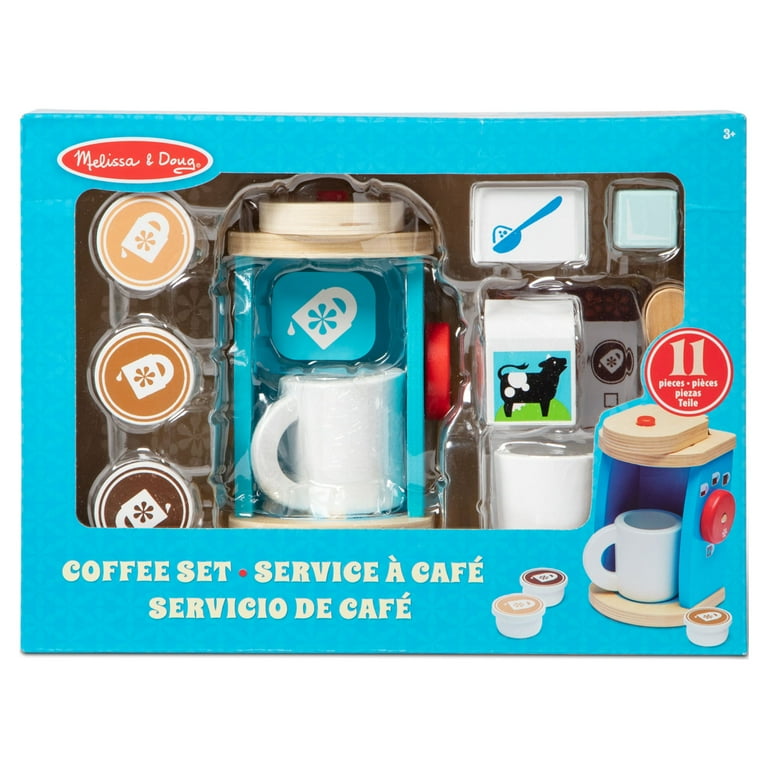This photograph showcases a children's toy coffee set encased in a light blue box with a clear plastic window at the center, allowing a view of the contents. The top left corner of the box features a horizontal red oval with a white border bearing the brand name "Melissa and Doug" in white cursive lettering. In the top right corner, the age recommendation "3+" is clearly marked. The set includes a bright blue pretend coffee maker with light wooden accents and a bright red circle on the right side. Positioned underneath the coffee maker is a white mug. To the left, the package displays three pretend coffee pods ranging in color from light tan to dark brown, arranged in a vertical column. On the right side, the set includes a white canister for sugar, a wooden spoon, and a light blue cube symbolizing milk. The bottom of the box prominently states "Coffee Set," followed by the translations "Service A Cafe" and "Servicio De Cafe" separated by a red dot. An additional image on the right side of the box illustrates the coffee set in action, highlighting its interactive elements.